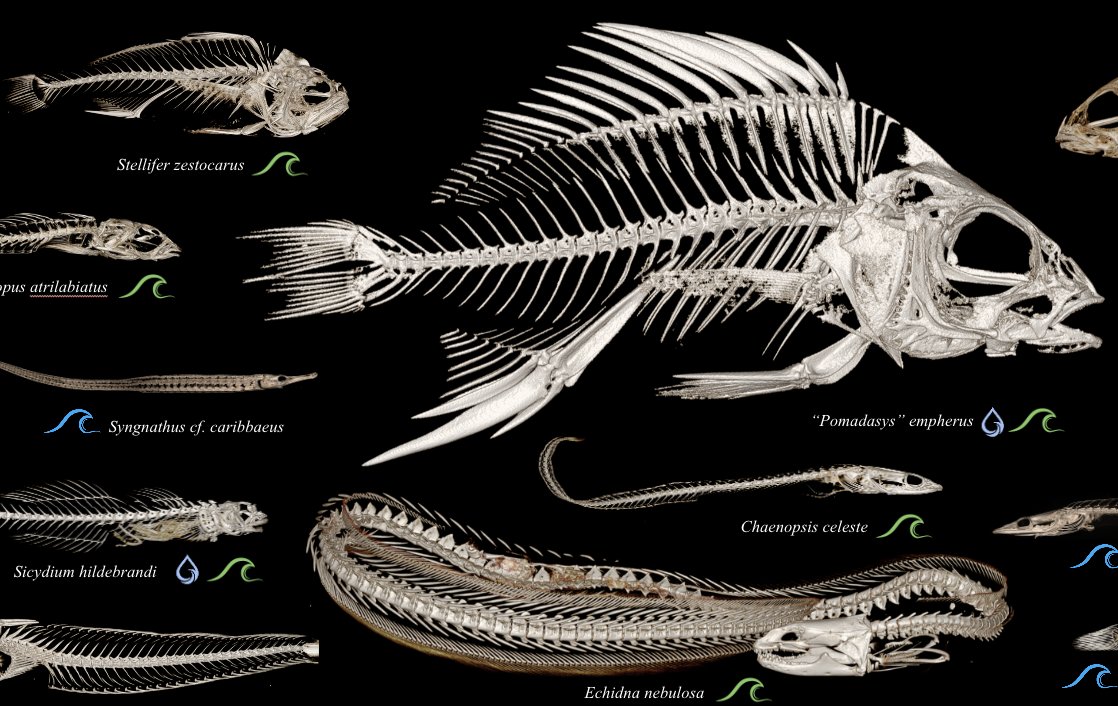The image features an array of meticulously detailed artistic renderings of various fish skeletons, set against a black background for a striking contrast. The skeletons, all labeled with their scientific names, predominantly face to the right, although some in the right corner point to the left. At the top left, we have three small skeletons stacked vertically: Stellifer zetocarus, Atrilabias, and Syngagnatus c.f. carabias. Below them are two more small skeletons, Psychidium hildebrandi, followed by an unnamed skeleton.

Dominating the right side is a very large skeleton labeled Pommadesus amphirus. Beneath it is a smaller skeleton of Chaenopsis cellist, and a notably long and large skeleton named Echidna nebulosa. Each fish skeleton is accompanied by icons—green and blue wave symbols, with one featuring a unique purple teardrop and green wave combination—possibly indicating their aquatic environments. The detailed skeletal representations capture the intricate bone structures, devoid of any muscles or skin, presenting an informative and visually engaging chart.